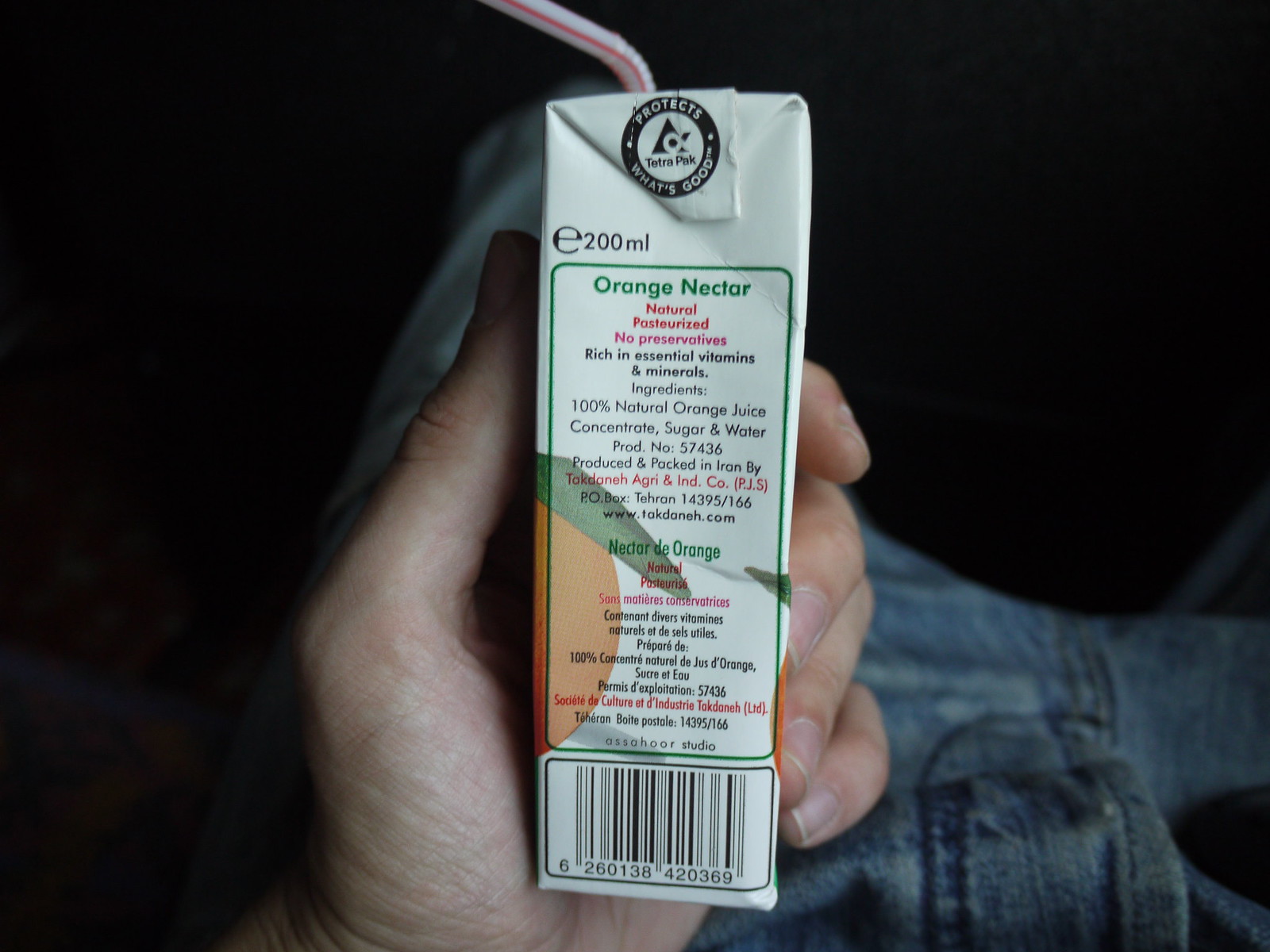In this image, you are looking down from the perspective of someone holding a 200 milliliter juice box labeled "Orange Nectar." The juice box is white with mostly black text and some red and green accents. It features a red and white striped, bendable straw sticking out of the top, and prominently displays a circular environmental design in black and white. The text on the box details that it is natural pasteurized, contains no preservatives, and is rich in essential vitamins and minerals. Ingredients listed include 100% natural orange juice concentrate, sugar, and water. A barcode with the numbers 261, 266, 138, 420, 369 is visible at the very bottom, along with a product number 57 436. The hand holding the juice box is a left hand, appearing to belong to a person of European descent who is wearing light denim jeans, visible below the juice box, against a black background.